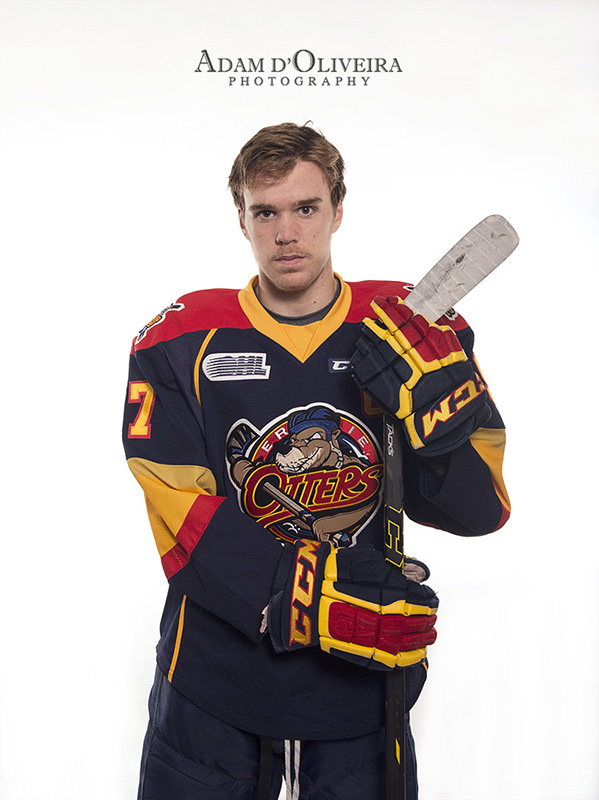The image depicts a professional male hockey player standing against a plain white background, which prominently features the watermark "Adam D. Oliveira Photography" at the top. The player is a young white male with reddish-brown hair and a trace of a mustache, staring straight ahead with a serious, emotionless expression. He is dressed in a dark blue hockey uniform with red shoulders and yellow trim. The jersey prominently displays the team's mascot, an otter wearing a blue hat, within a circle on his chest, and the word "Otters" in bold red letters. He is wearing large hockey mittens matching the uniform's color scheme of blue, yellow, and red, and is also holding a white hockey stick.